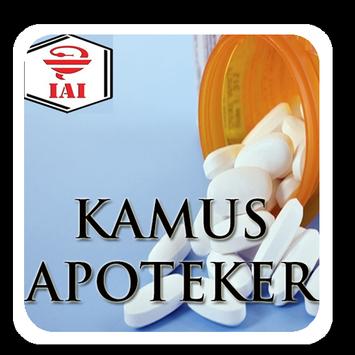The image depicts an advertisement for a pharmaceutical company, featuring a black background with a squared-off border. Central to the image is a rounded white square outline, framing the main visual elements. In the upper right-hand quadrant, there is a close-up of the top of an orangey-brown pill bottle from which 15 to 20 oval-shaped, unmarked white capsules are spilling out, resembling a horn of plenty. The background within the white outline is a lighter blue, creating contrast with the black border. In the upper left-hand corner, a hexagonal label houses a red logo that has the initials "IAI" with some sort of abstract red design, possibly evoking a mortar and pestle. Below the image of the pills, there is black lettering that spells out "KAMUSAPOTEKER," suggesting a word related to apothecaries or pharmacists.